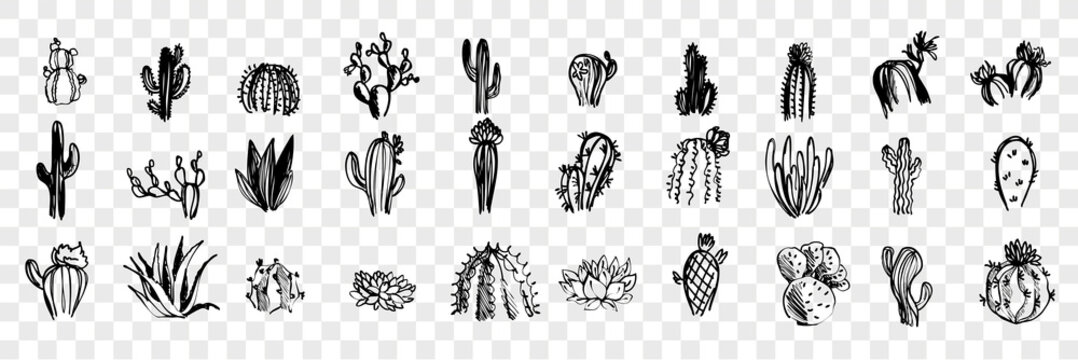This image features a series of 30 distinct black-and-white line drawings of various cacti, organized neatly into a 3-by-10 grid. Each drawing captures a different species or variation of cacti, showcasing a range of forms from traditional, multi-branched types to round and grass-like shapes. The illustrations are rendered in a graphic or clip art style without any ground roots, focusing instead on the stems and, in some cases, the prevalent spikes. The background is a light gray and white checkerboard pattern, reminiscent of a transparent background in digital image editing software, creating a uniform backdrop that highlights the detailed line work of each cactus drawing.